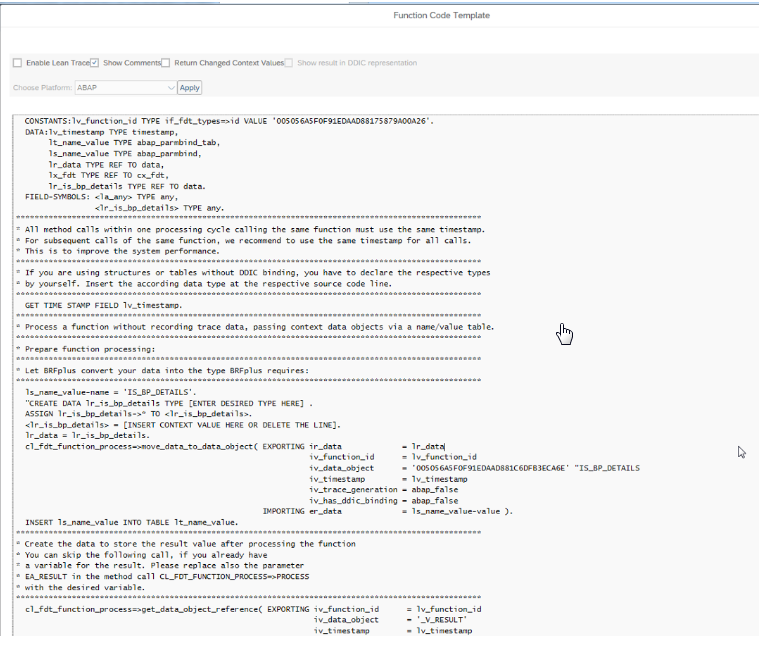At the top of this web page, a prominent blue line stretches horizontally from left to right. Centered beneath this line in bold, black letters, the phrase "Function Code Template" stands out. Directly above this title is a thin, gray rectangle containing several checkboxes with labels beside them:

1. "Enable Lean Trace"
2. "Show COM Something" (with a blue checkmark)
3. "Return Charged Convert Value"
4. "ABAP" and "Apply"

Below "Function Code Template" lies a large gray rectangle, featuring a significant amount of black text. The text is printed on a gray background, making it hard to read. Within this rectangle, the text appears structured into paragraphs, each separated by a horizontal line formed of dotted lines. 

The first section lists:
- "Constants"
- "Data" followed by "Name," "Value," "Type"

Subsequent sections contain:
- "A11 Method within one processing cycle"
- "If you're using Structure or Tables without DOIC Binding"
- "Get TDE Field"
- "Process a Function without Recording"
- "Prepare Function Processing"
- "Let BBF Plus Convert Your Data"
- "Insert, Create. You can skip the following call if you already have it."

Additionally, there are several other pieces of text that are too small to read, even with assistance from magnifying glasses ("cheater glasses"). The entire layout of the page appears dense and information-laden, posing a challenge for clear and easy readability.